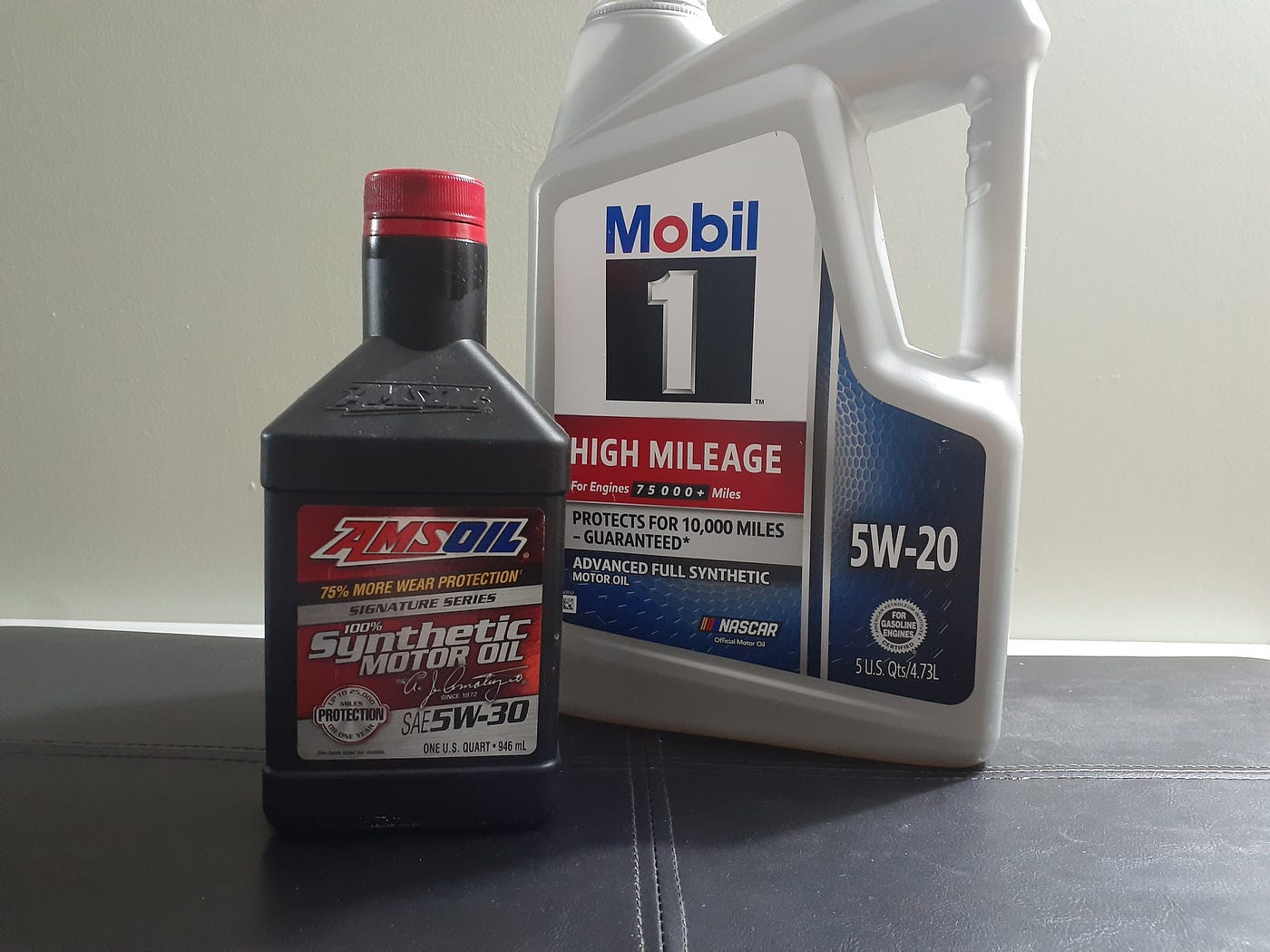The image features two automotive products placed on a dark linoleum floor against a white or off-white background with white molding. On the right side, there's a large, white, 5-liter container of Mobil 1 High Mileage motor oil. The bottle has a distinct design with the 'Mobil 1' logo at the top, featuring 'Mobil' in blue and red letters and a black box with a white number '1'. Below, a red bar highlights 'High Mileage' in white font, and beneath it, in gray font, it reads 'Advanced Full Synthetic'. A blue, dotted pattern displays '5W-20' alongside a small logo and additional product details.

On the left, there's a smaller black bottle with a red cap labeled 'AMSOIL Signature Series', embossed with 'AMSOIL' in red and blue lettering. It prominently advertises '75% More Wear Protection' in silver lettering. The label indicates that it is a '100% Synthetic Motor Oil, SAE 5W-30' with further details in white font over a red and gray background. Both products are designed for different purposes in automotive maintenance.